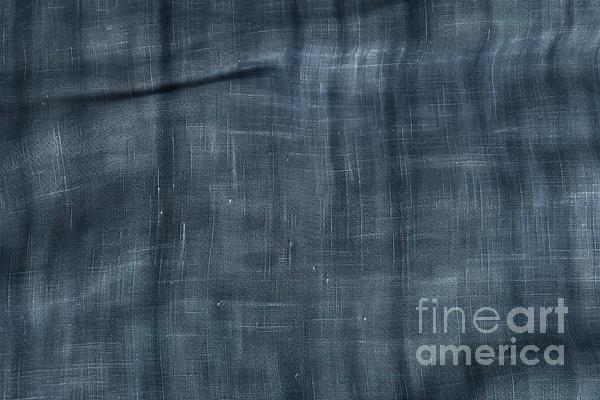The image is a detailed close-up of a well-worn, blueish-gray fabric, likely a tablecloth, that features delicate variations in its texture. The fabric has a weathered look, with a blend of several blue shades, ranging from dark blue to nearly white, forming fine lines that run both vertically and horizontally across its surface. These lines might be the result of underlying threads showing through, giving the fabric a distinct, slightly textured linen appearance. Scattered throughout the fabric are subtle folds and permanent creases, indicating years of use and appreciation. In the top left corner, a significant fold marks the fabric, suggesting it has been crushed or bent over time. In the bottom right corner, there is a gray, semi-transparent watermark that reads "Fine Art America," with the word "fine" in a thin font, and "art" and "America" in a thicker weight, all in lowercase lettering.